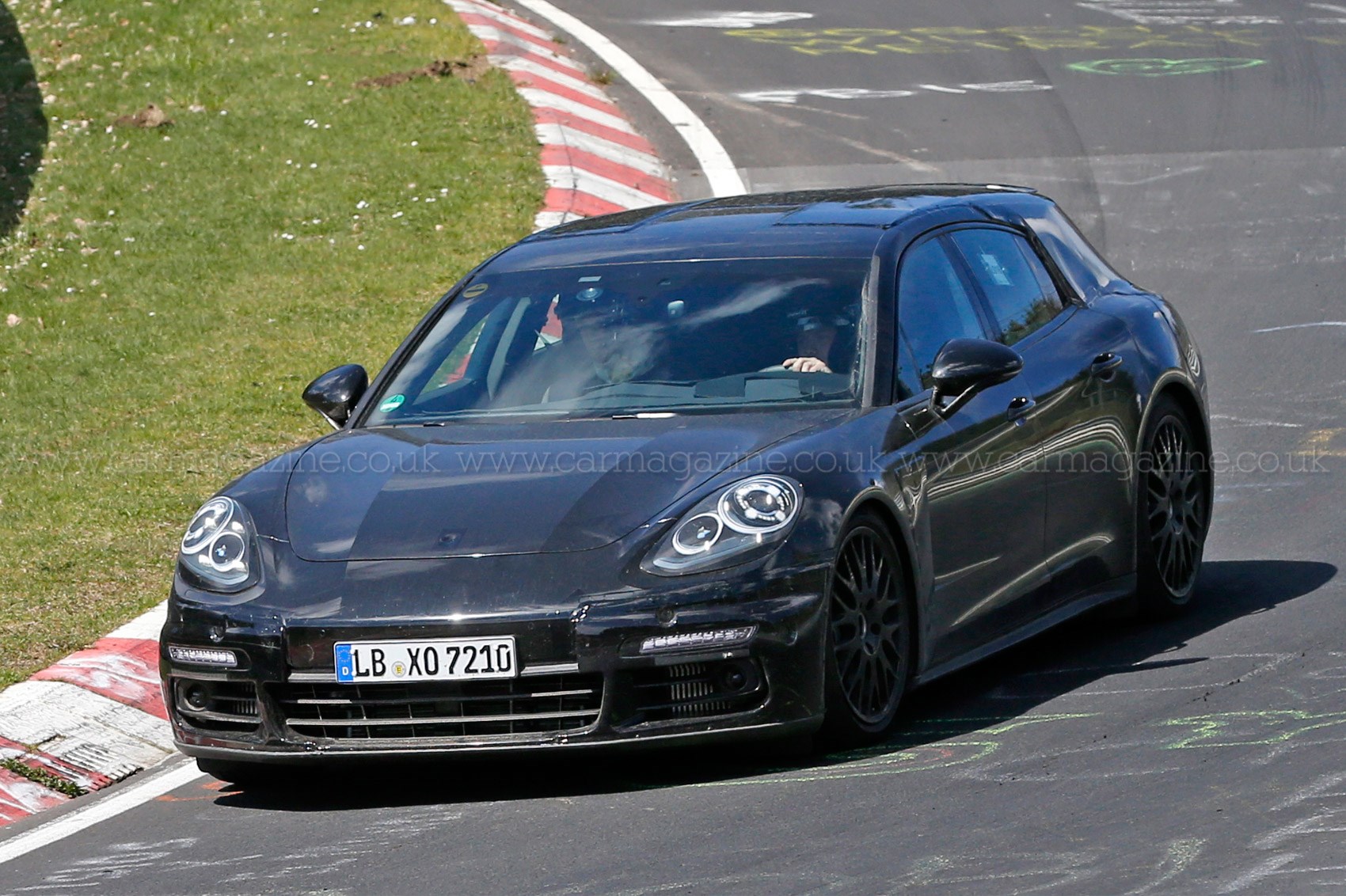In this realistic, horizontally-oriented photograph taken during the day, the scene is well-lit and sunny. The image captures a black, sporty, four-door car with a low-to-the-ground profile and four headlights, navigating a turn on a racetrack. The racetrack is dark gray asphalt, curving in a backwards ‘C’ shape as viewed from the angle of the photo. The car's front license plate reads "LBX07210" in black text on a white background. To the left of the track is a strip of green grass, likely forming the median, bordered by a red and white striped barrier commonly seen at the edges of racetracks. The car, which appears to have a driver whose hand and part of their neck are visible, is positioned in the center of the image, emphasizing its dynamic movement around the curve.